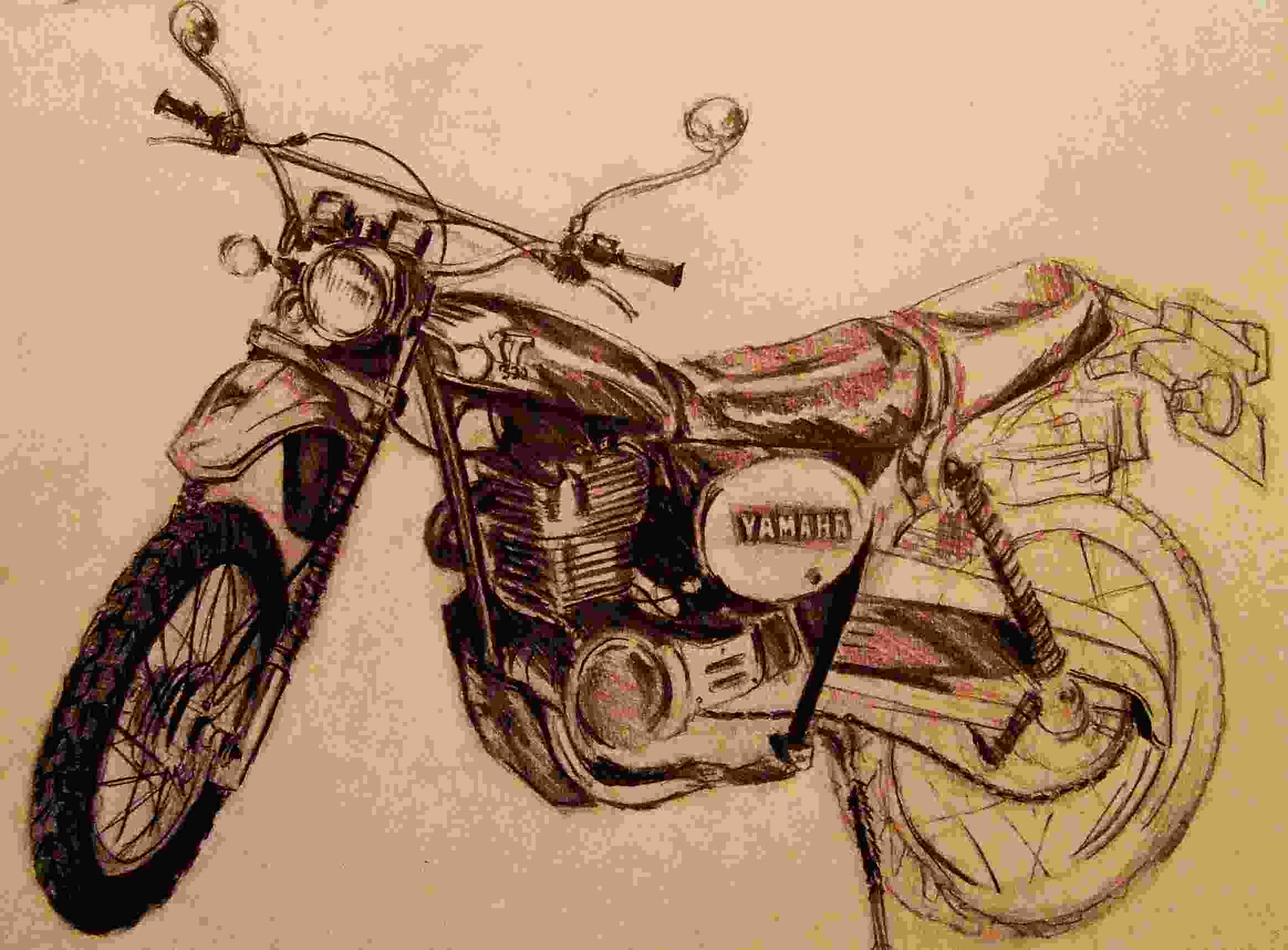This image depicts a detailed sketch of a Yamaha motorcycle, prominently displayed against a pale pink and gray, or possibly peach, vector-like background. The illustration appears to be rendered with colored pencils or ink, featuring smooth lines with a noticeable texture that one would associate with traditional sketching mediums. The motorcycle fills most of the space in the image and is viewed from the side, with the front tire and handlebars turned outward. 

The front end of the motorcycle, including the headlight, small tire, straight handlebars, and noticeable mirrors, is thoroughly detailed and richly colored, featuring red embellishments that resemble a blood red or rust brown hue. The engine and the "Yamaha" plaque are also clearly visible and well-defined. However, the drawing transitions to a less finished state towards the rear of the bike. The back tire, rear bumper, rear brake lights, and the area beneath and behind the two-seater seat remain as simple outlines without color or detailed shading. This incomplete section contrasts with the meticulously finished front, emphasizing the work-in-progress nature of the artwork.